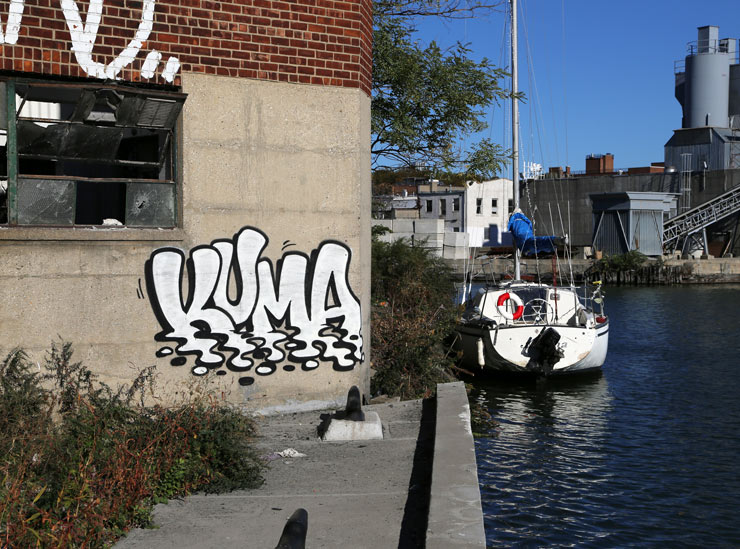This outdoor daytime photograph, measuring approximately five inches wide and four inches high, captures a rundown industrial area. Dominating the right half of the image is a blue water canal with a white sailboat, its sail wrapped up and a black motor visibly mounted on the rear. The boat is docked, and above it lies a strikingly blue sky that contrasts with the gray, factory-like buildings which carry an industrial and somewhat neglected appearance. The water in the canal is a dark blue, almost black hue.

The left half of the image features a gray cement walkway at the bottom, leading up to a decrepit stone building constructed from large cement stones at the base and red bricks on the upper portion. This building has a broken window on the left side, with a piece of white graffiti reading "Kuma" outlined in black located in the lower right corner of the window. Red and green weeds grow from the walkway, adding to the scene’s abandoned aesthetic. The overall atmosphere conveyed by the photograph is of industrial decay and subtle urban neglect.